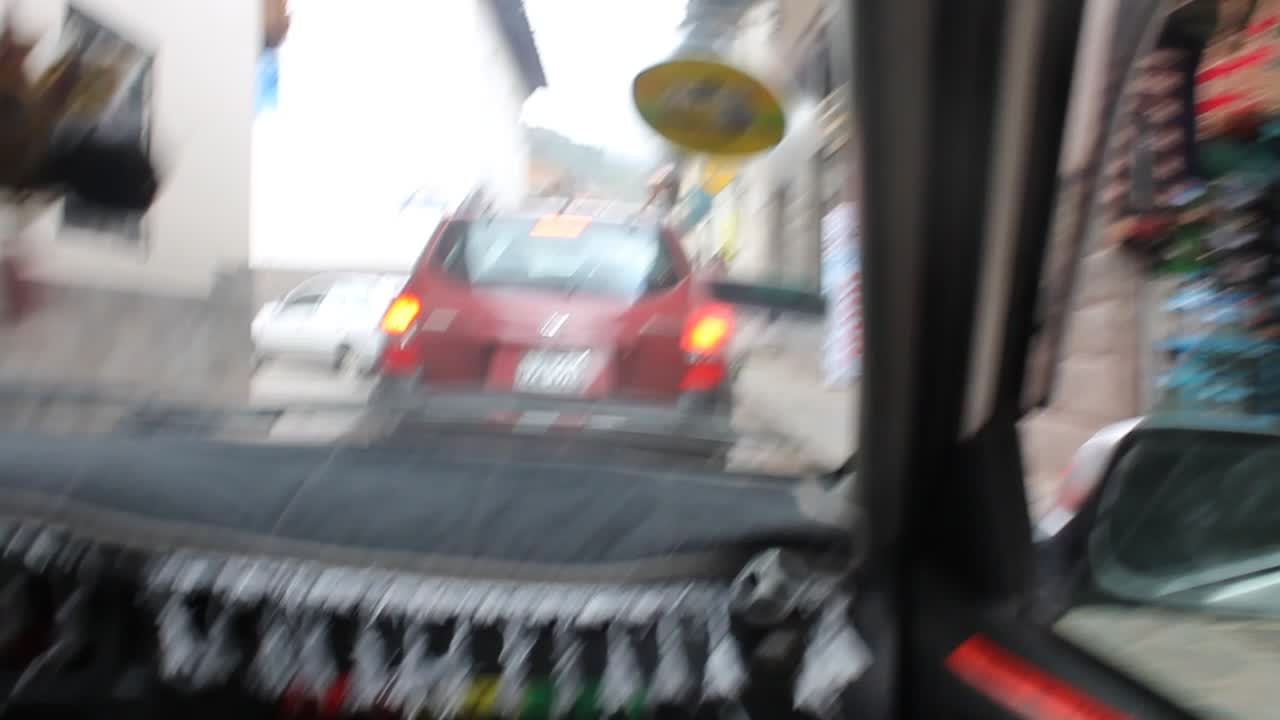This blurred image, presumably taken from the passenger seat of an American-style vehicle, captures a scene through the windshield and side window. Draped across the dashboard is a cloth cover adorned with tassels. Directly ahead is a red SUV with a gray bumper, its brake lights glowing. The right side of the frame includes the vehicle's window edge and side mirror. Alongside the vehicle, near the street edge, several colorful buildings come into view. One building in particular stands out, possibly a storefront displaying vibrant products, hinting at a bustling or commercial area.